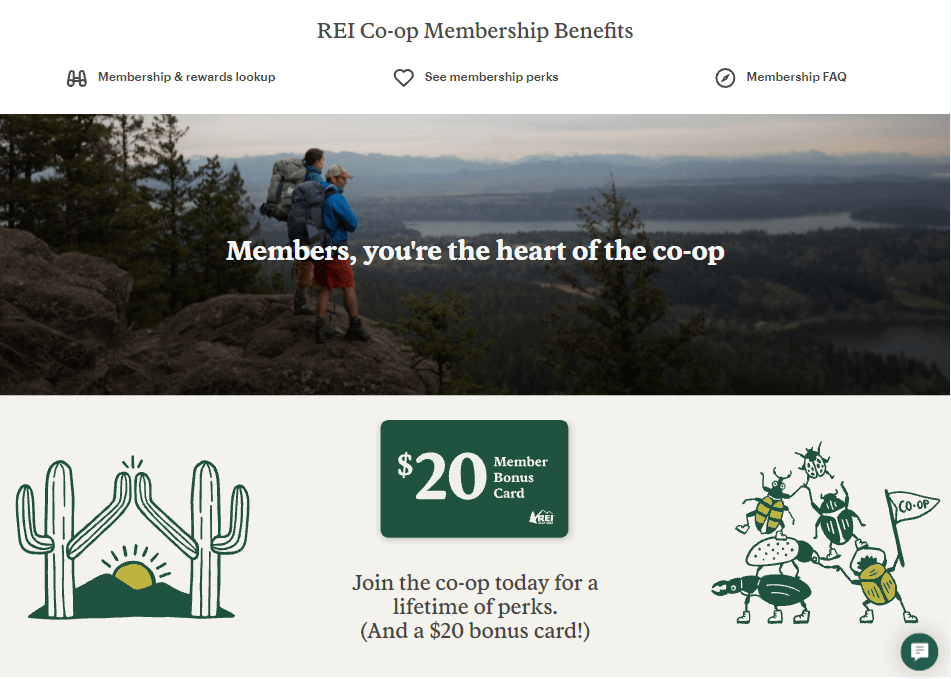The image is a screenshot taken from a computer displaying the "REI Co-op Membership Benefits" page. At the top of the page, the title "REI Co-op Membership Benefits" is prominently shown, with "REI" in all capital letters. To the left, there's a section labeled "Membership and Rewards Lookup," followed by "See Membership Perks." On the far right, there is a link for "Membership FAQ."

In the middle of the page, a captivating photograph depicts a group of hikers standing at the edge of a cliff. They appear to be enjoying either a sunrise or sunset, although the sky is hazy and overcast, obscuring a clear view of the sun. The hikers are equipped with backpacks, hats, shorts, and lightweight coats, suggesting they are prepared for varying outdoor conditions. Superimposed over this image is the text, "Members, you're the heart of the co-op."

The bottom section of the page features a whimsical illustration of cactuses high-fiving each other as the sun rises behind them. Accompanying this illustration is a clickable area that offers a "$20 Member Bonus Card." To the right of this, several cartoon bugs are visible, holding a flag that reads "Co-op," adding a playful touch to the page's design.